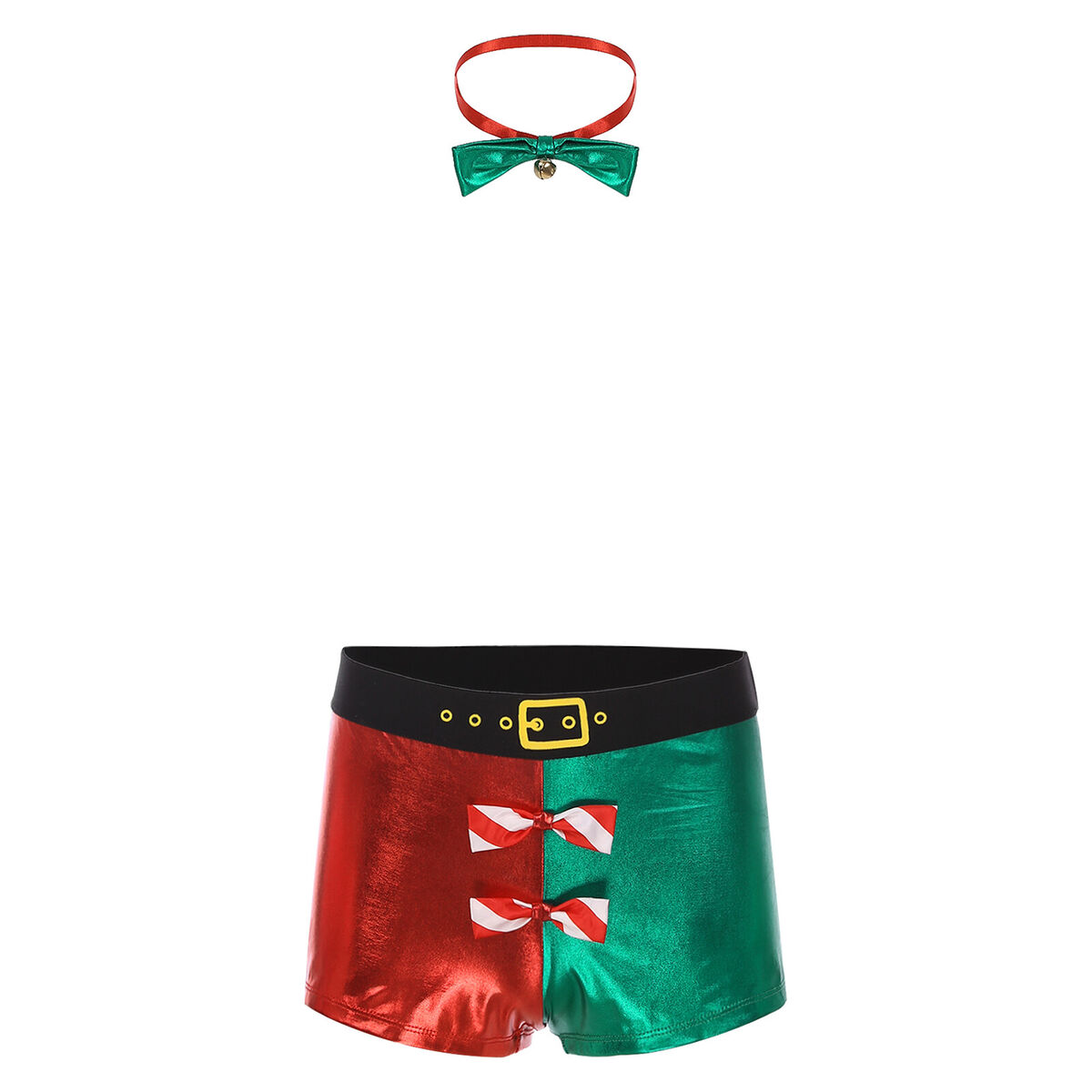The image features two distinct items against a white background, both of which are evidently designed for a Christmas-themed costume. At the top is a red collar adorned with a green metallic bow and a small gold bell hanging in the middle, giving it a festive holiday look. Below the collar, approximately eight centimeters apart, is a pair of silky men's boxer shorts. The shorts, made from a satin-like material, are divided into two vibrant halves: one side is red and the other is green, both hues possessing a metallic sheen. A faux black belt with a gold buckle runs around the top of the shorts, reminiscent of Santa Claus's iconic attire. Two candy cane striped bows, in red and white, are centrally placed just underneath the belt buckle. Overall, the ensemble appears to be a playful and risque Christmas costume set perfect for a festive holiday party.